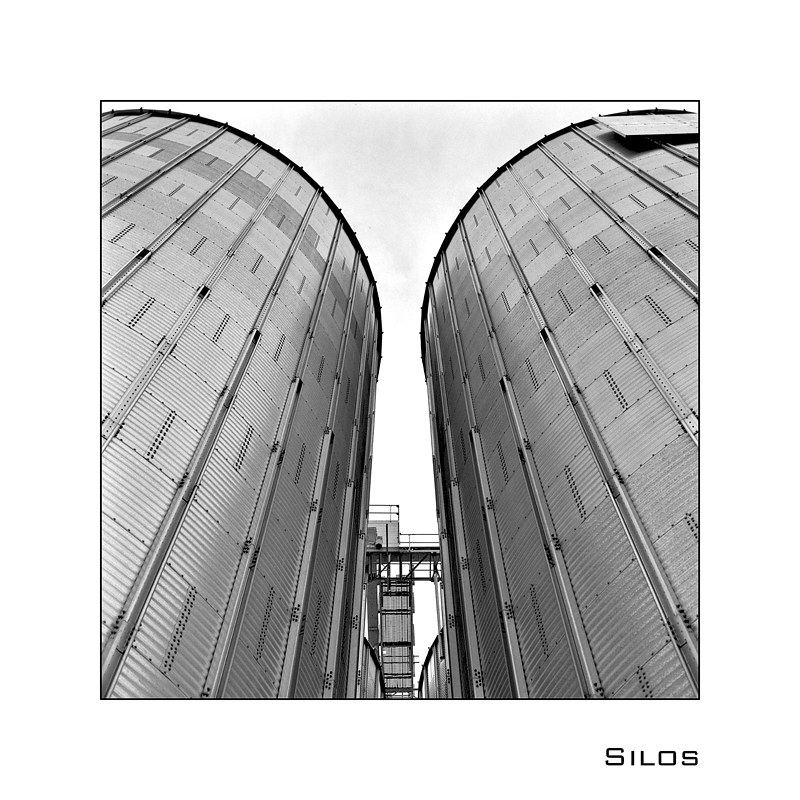This black-and-white photograph, taken from a low angle, captures the imposing presence of two extremely tall, light-colored silos. These silos, braced with multiple panels of corrugated metal and stiff support ridges, converge towards the center of the image due to the perspective of the shot. Connecting the towering structures is a catwalk-style bridge, high above the ground, that provides a functional link between the silos or possibly other metal buildings. In the lower right corner, on a white background, the word "Silos" is prominently displayed in gray. The overall scene exudes a sense of newness and structural integrity, set against a monochromatic, possibly gloomy, sky.